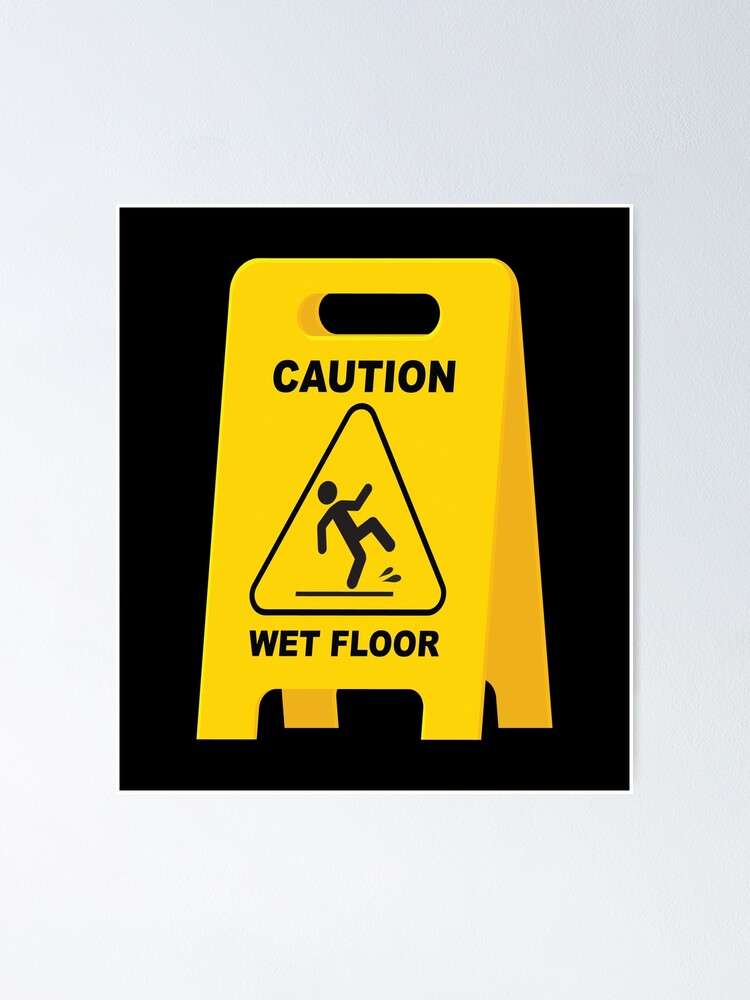The image features a yellow caution wet floor sign set against a black square background, itself bordered by a thin white trim. The yellow sign, commonly seen in industrial office buildings and stores to warn of slippery conditions, is depicted center-stage. The sign stands vertically with its four-leg base and a handle at the top for easy transport and collapsing. The caution sign is prominently marked with a black triangle containing a stick figure slipping backward, with one leg lifted off the floor and two large water droplets beneath it to indicate the hazardous wet floor. Above the triangle, the word "Caution" is displayed in black text, and below it, "Wet Floor" is also written in black lettering. The image is simplistic yet effective in its communication, utilizing common visual cues to ensure the message is clear and readily understandable.